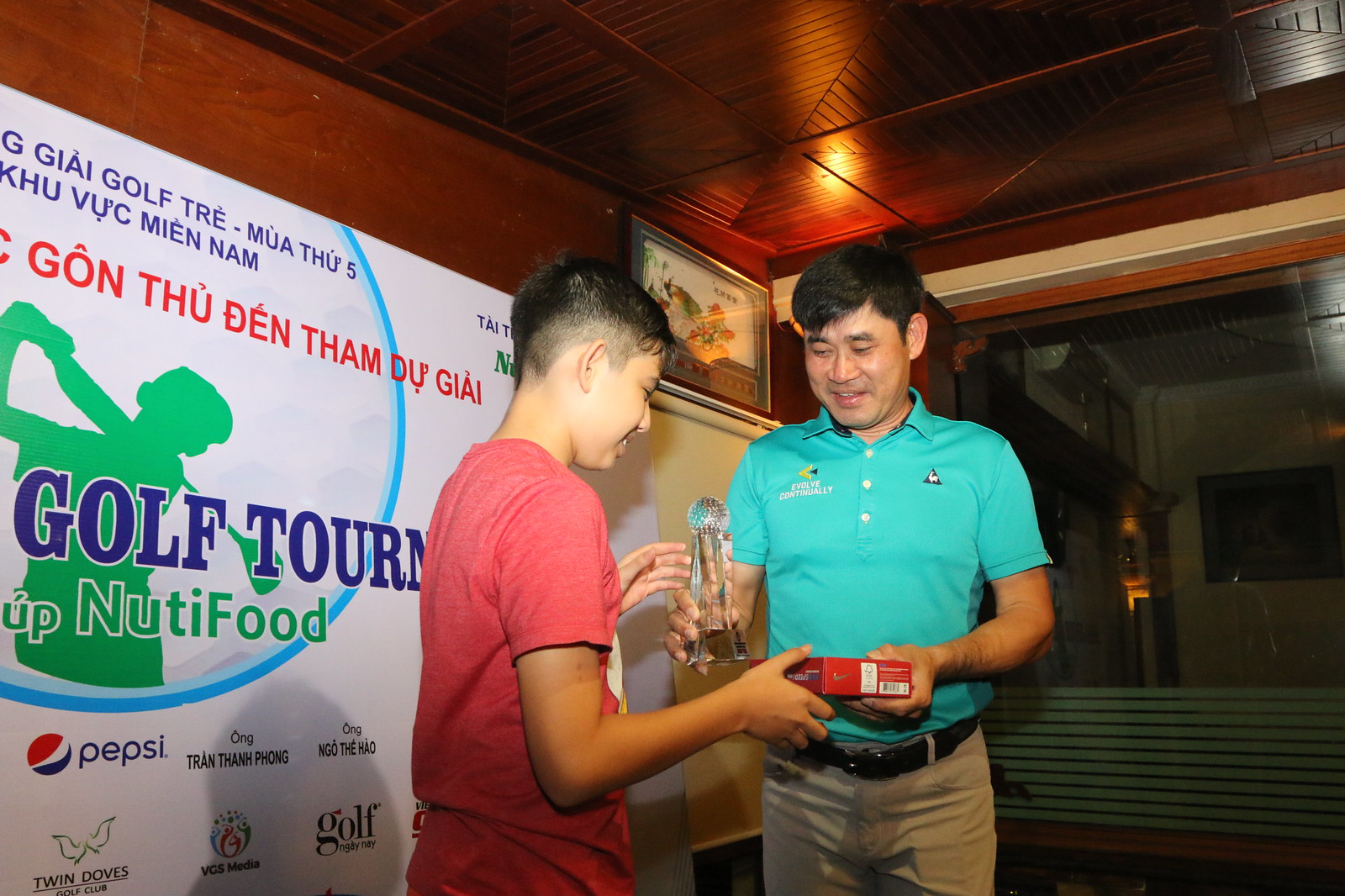The image depicts an indoor scene at night, likely taking place in the corner of a room or a hallway, characterized by the redwood-style ceiling and visible brown, white, purple, red, green, light blue, black, orange, and pink colors. Positioned centrally in the photograph, a man of Asian descent, possibly Vietnamese, is seen presenting a young teenage boy, also of Asian descent, with two items: a glass cylindrical trophy topped with a golf ball, and a red box with a Nike logo. The man, dressed in a light teal short-sleeve polo shirt and khaki pants with a belt, has short black hair and appears to be mid-sentence, his arms bent at the elbows as he hands over the items. The teenage boy, sporting a short faded haircut, is wearing a short-sleeve red t-shirt, arms also bent at the elbows ready to receive the awards. Behind them is a large white banner featuring an image of a person swinging a golf club, and text primarily in Vietnamese, save for the blue "golf tournament" caption. The wall also displays logos of sponsors such as Pepsi and Twin Doves. To the right side of the image, a window is visible, indicating the darkness outside. The setting seems to be an award presentation, celebrating a golf event.